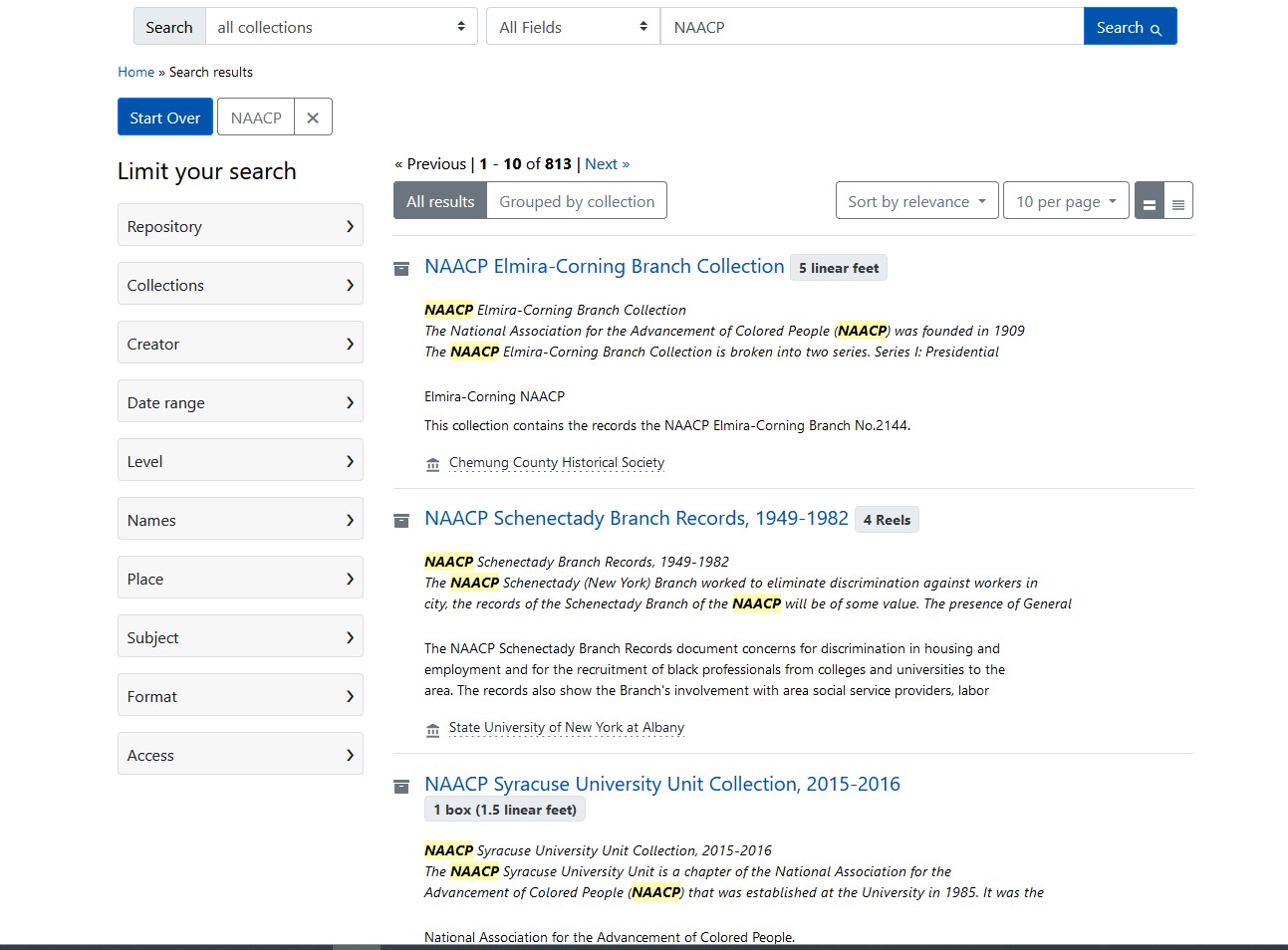In this detailed photographic image of a web page, the interface presents a comprehensive search feature. At the very top, we see a gray search bar labeled "All Collections" accompanied by up and down arrows. Below, there is a primary search bar with a magnifying glass icon encased in a blue button. Within this search bar, the term "NAACP" has been entered. Below this, the navigation bar features a blue 'Home' button, followed by the words "Search Results" in black, and a blue 'Start Over' button. To the right of "NAACP" in the search bar, there is an 'X' icon for clearing the search term.

The page is organized with several filtering options labeled "Limit Your Search," "Repository," "Collections," "Creator," "Date Range," "Level," "Names," "Place," "Subject," "Format," and "Access," each with an arrow to the right indicating further selection is available. Below these filters are search results in the form of hyperlinks. The highlighted collections include the "NAACP Elmira Corning Branch Collection," the "NAACP Branch Records, Schenectady, 1949-1982," and the "NAACP Syracuse University Unit Collection, 2015-2016." The page design is user-friendly, offering structured navigation and detailed search functionality for exploring NAACP records.